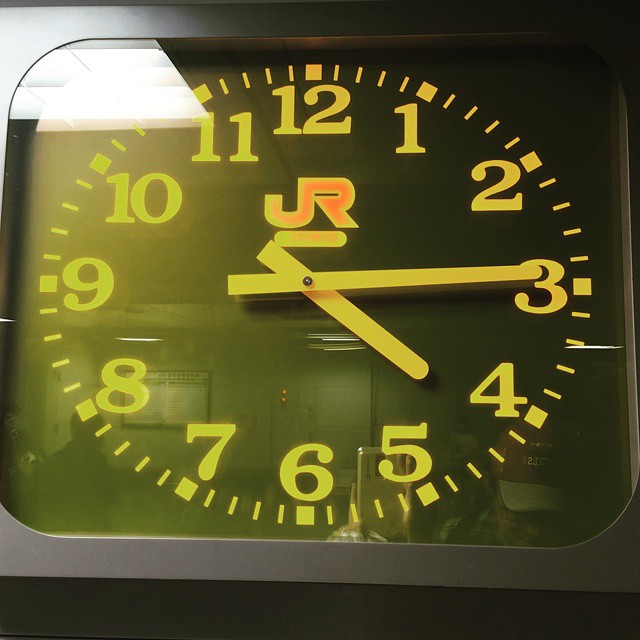This close-up image captures a square alarm clock with rounded corners, set against a brown wooden desk. The clock's frame is thin and brown with a clear plastic lens over the face, which is also brown, creating a 3D effect with the recessed face. The analog clock displays the time 4:15 with yellow numbers and short segmented lines marking the minutes. The hour markers are small squares, and both the hour and minute hands are yellow, designed like popsicle sticks on one end and square on the other. The clock bears the label "UR" or possibly "JR," underlined above the center in pinkish letters with a yellow outline. A shiny surface of the clock reflects an image from the room, showing an older man wearing a red and gray baseball cap, black-framed eyeglasses, and a flannel shirt. In the reflection, another man is visible to the left, and various other details, including fluorescent white light, a doorway, and a horizontal item with a black frame hanging on the wall, are also discernible.